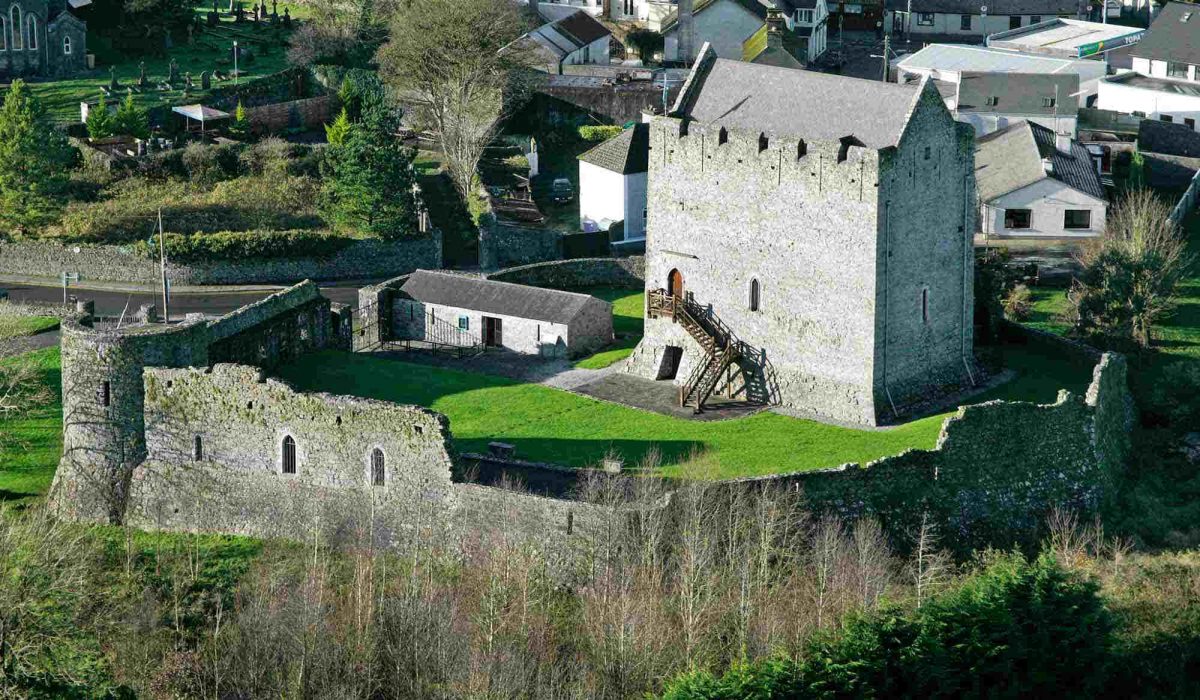The image depicts the remnants of a historic stone castle, encircled by a partially deteriorated rock wall with arched windows and turrets prominently visible on the left side. Central to the picture is a multi-story stone house, protected within the fortress. This grand house features a distinctive stairway ascending to the second floor, where a lone window faces forward. Additional windows punctuate the house's side, contrasting with the largely windowless lower floors. 

Adjacent to the house is a smaller guardhouse-like structure with a gate connecting it to the main road. The lush, vibrant green lawn enhances the castle's majestic appearance. The surrounding scenery reveals numerous modern houses with varied roofing, as well as scattered trees in the foreground and background. A mix of single and double-story homes, along with overarching greenery, adds to the picturesque setting. Despite signs of decay, including some broken sections, the historic fortress and its central house remain imposing and evocative.